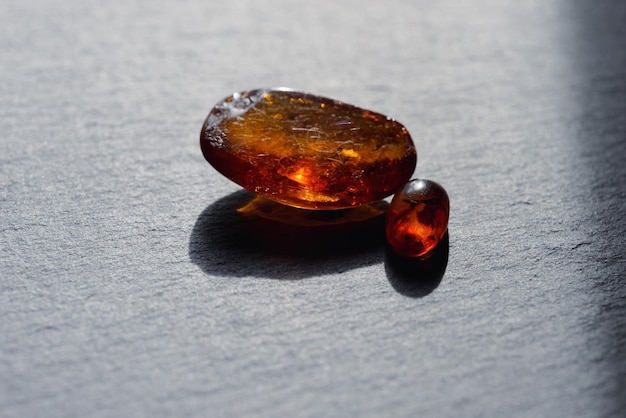The image depicts two amber-colored oval objects, set against a gray background. The larger of the two objects, which lies horizontally, has a more intense and varied orange hue with hints of gold and a rougher texture. This object also features a brighter orange spot in the center and appears to be more pill-shaped. The smaller object, positioned vertically to the right of the larger one, shares a similar brownish-gold color with lighter shades but is noticeably smoother. Both objects cast shadows on the gray surface beneath them, adding depth to the composition and highlighting their shapes and textures. The interplay of light illuminates different shades within the objects, suggesting they could be gemstones or man-made items with a pill-like appearance.